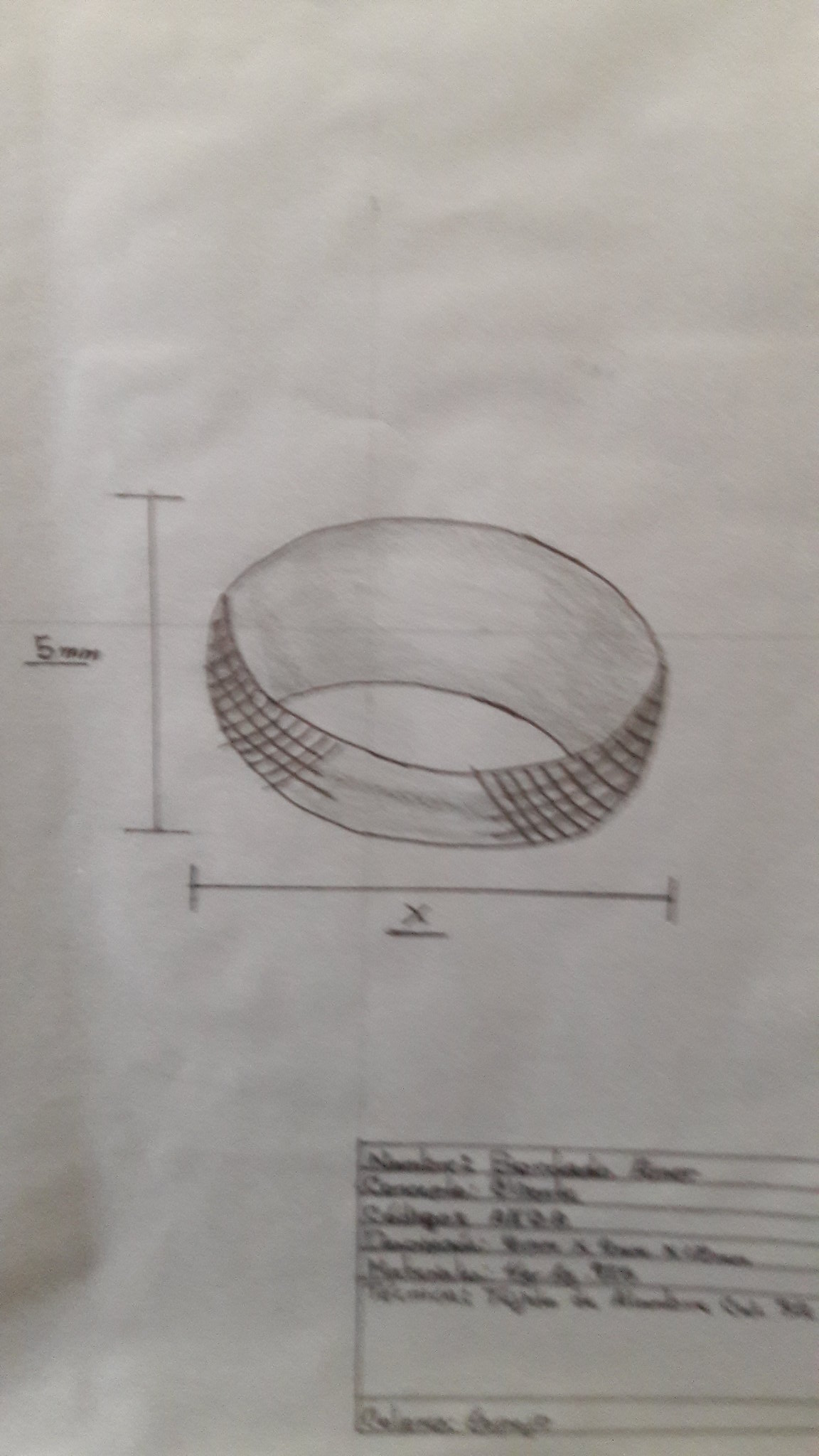**Detailed Caption:**

This image features a detailed pencil drawing on a white sheet of paper. Central to the drawing is a cylindrical object, resembling a bracelet, depicted with its round shape and visible interior. The outer surface of the object is adorned with intricate checkerboard patterns, except for a distinct white section that lacks these patterns. 

To the left of this section, a vertical bar resembling a tall "I" extends from the top to the bottom of the drawing, likely indicating the dimensions of the cylindrical object. Accompanying this bar is some text that is too small and indistinct to be read clearly. Similarly, at the bottom of the cylindrical object, another bar appears, marked with an “X,” also suggesting measurements. Below this bar, there is additional text, but it remains indecipherable due to its blurriness.